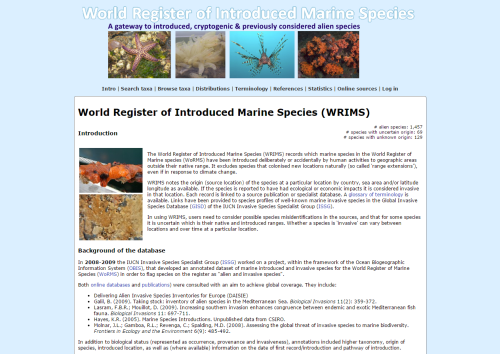A detailed caption for the image could be:

"The screenshot captures an information page titled 'World Register of Introduced Marine Species.' At the top of the page, the title is prominently displayed along with a tagline that reads 'A Gateway to Introduced Cryptogenic and Previously Considered Alien Species.' Below the main heading, the content indicates that the page belongs to the 'World Register of Introduced Marine Species (WRIMS).' The section titled 'Introduction' appears to provide an overview of the database and its purpose, though the text within the paragraphs is too small to read clearly. One of the visible subtitles is 'Background of the Database,' likely offering detailed information on the database's origins, objectives, and the scope of the information it provides about marine species that have been introduced to new environments."